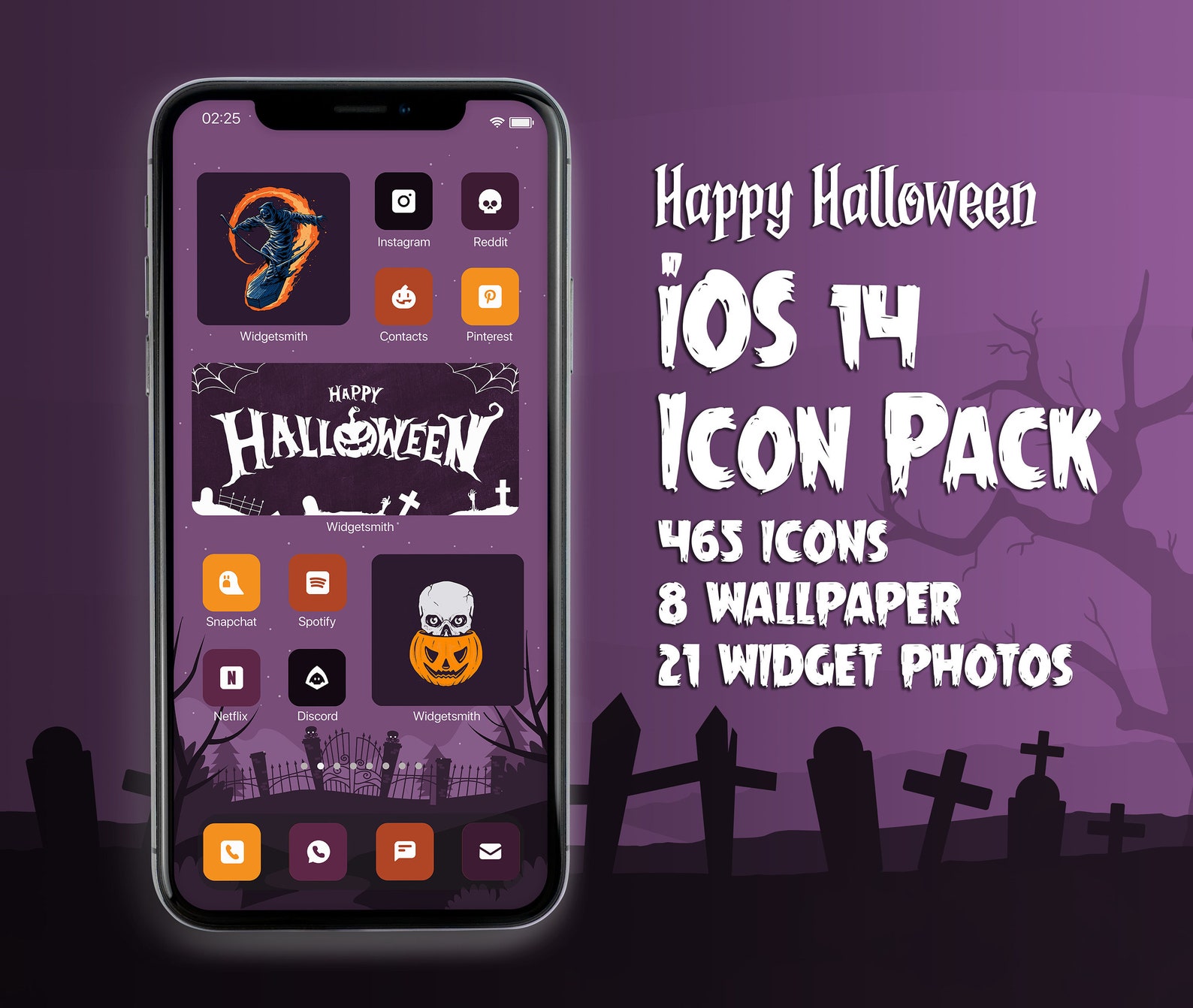A vibrant Halloween-themed advertisement set against a striking purple, lighter purple, and black gradient background showcases an iOS 14 icon pack. The ad, with a distinct "Happy Halloween" title in a weathered white font, features a cell phone displaying the same festive theme. The screen shows an array of Halloween-styled widgets and app icons, including a mummy and icons for popular apps like Instagram, Reddit, Contacts, Pinterest, Widget Smith, Spotify, Discord, Netflix, and Snapchat. Notably, some app icons are transformed to fit the spooky theme, such as the Reddit icon now featuring a skull instead of the usual alien mascot.

The phone’s display and the backdrop both depict an eerie gray sky fading into a gray yard, filled with silhouettes of crosses, tombstones, and a barren tree on the right side, enhancing the Halloween atmosphere. The icon pack includes 465 unique icons, 8 wallpapers, and 21 widget photos, providing a comprehensive and cohesive spooky aesthetic for the user's device.